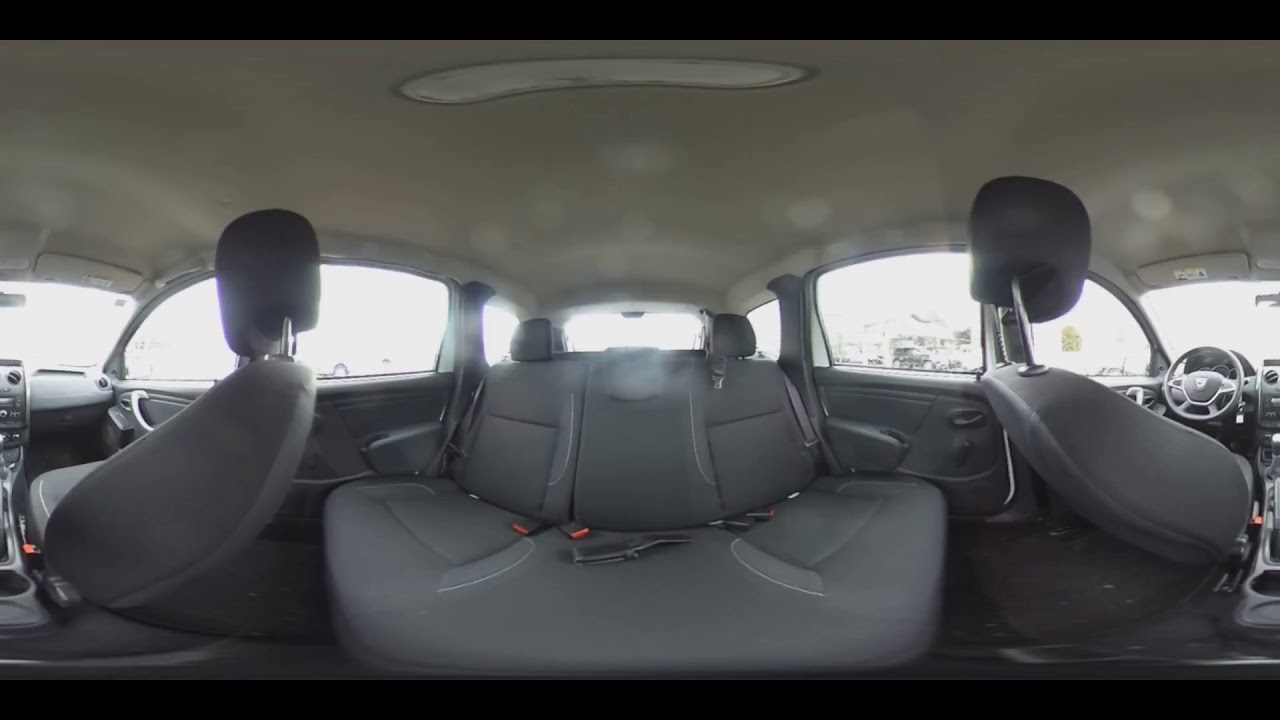This panoramic, fisheye view photograph captures the clean, pristine interior of a car, showcasing its detailed features. The car seats, made from a decent gray fabric (not leather), are spotless and arranged to fit four to five passengers comfortably. Visible are the front seats with headrests pulled up high, the driver's seat, and the empty backseat, ensuring the car's spaciousness is evident. The interior's accents include orange seatbelts and red safety belt clips. At the center top of the beige headliner, there is a dome light illuminating the gray interior. Notable elements include a gray steering wheel with silver accents, a positioned key on its right side, and traditional roll-up window handles. Through the clear glass windows, daylight brightens the inside, and a white building with a black jeep with silver alloy wheels parked in front can be seen outside. Ventilation grilles on the left side of the image further detail the car’s interior.